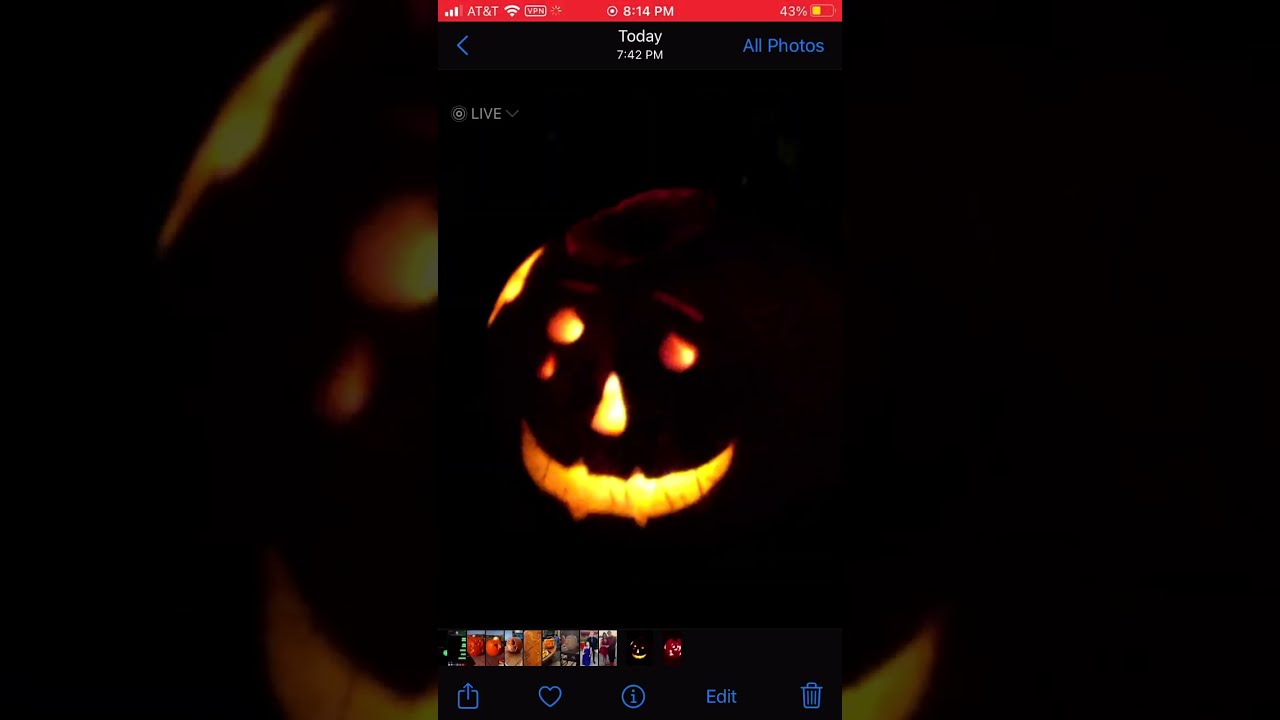The image is a vertical screenshot of a phone displaying a darkened interface, likely from a photo app. A prominent red bar at the top reads "AT&T" alongside icons indicating WiFi signal strength, the time (8:14 PM), and the battery level at 43% represented with a yellow battery icon. Encased in the center of the screen is an illuminated jack-o'-lantern, exhibiting two glowing eyes, a lit nose, and an orange-yellow mouth. Notably, a teardrop appears to be falling from the jack-o'-lantern's right eye, adding a unique feature. The image is bordered on the left and right by a blurred, enlarged portion of the jack-o'-lantern's image, serving as a decorative backdrop.

At the top left, the word "Live" is visible, while on the right, blue text notes "All Photos." Beneath the central image, a row of smaller preview images is barely discernible, adding context that the screenshot is from a photo browsing app. The lower portion of the interface displays a series of blue icons: from left to right, these include an upload arrow, a heart, an eye symbol within a circle, the word "Edit," and a trash can.